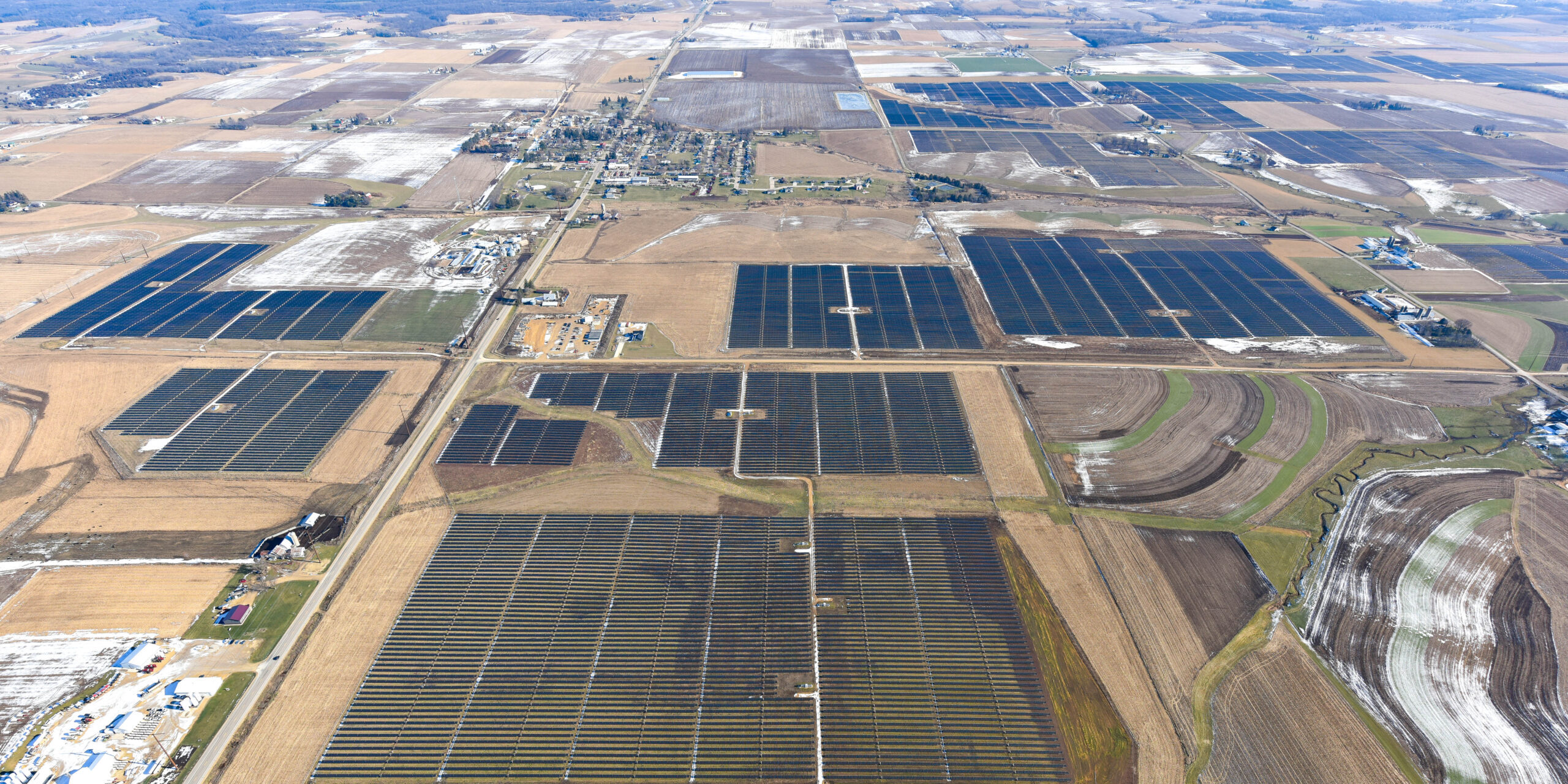The image is an aerial photograph taken during the daytime, capturing a large, intricately patterned landscape comprising predominantly farmland with a grid-like structure. The land is divided into numerous rectangular fields, reminiscent of rows of solar panels, though not all are uniformly rectangular or identical in size. These fields, varying in shades from green to beige, brown, black, and white, exhibit a very regular and orderly arrangement, suggesting active cultivation. The grids do not occupy the entire landscape uniformly; the bottom right corner features a terraced, stony landscape adding texture to the scene. Scattered small buildings, minuscule in comparison to the vast fields, suggest the presence of human activity. Towards the middle-left and the far-right edges of the image, a small town is visible, punctuating the predominantly agricultural expanse. The bright sunlight and clear outdoor visibility enhance the detailed and vibrant depiction of this rural expanse.